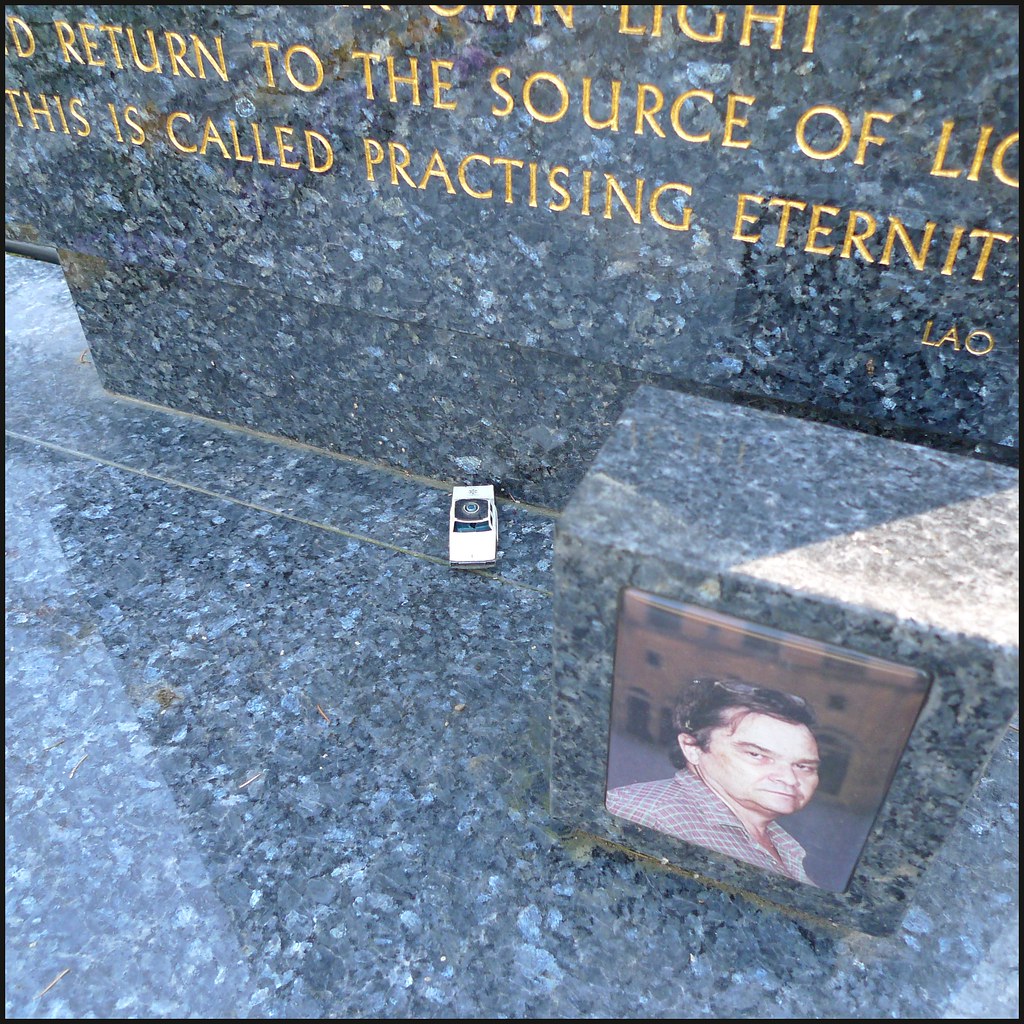The square image depicts a memorial statue or gravestone crafted from a striking grayish-blue, reflective marble material. The monument features a diagonal surface at the bottom, transitioning into an upright section adorned with gold text. The visible inscription reads, in all capital letters, "RETURN TO THE SOURCE OF LIGHT." Below this, a second line states, "This is called practicing eternity," with a smaller attribution reading "LAO" in the bottom right corner. Protruding from the bottom right is a rectangular block of the same marble, showcasing a photograph of a man with sunglasses perched on his head and brown hair. His expression appears to be a scowl directed towards the camera. To the side of this block is a small object, possibly a toy car, placed as part of the memorial. The overall composition strongly suggests that this is a tribute or gravesite dedicated to the man in the photograph.